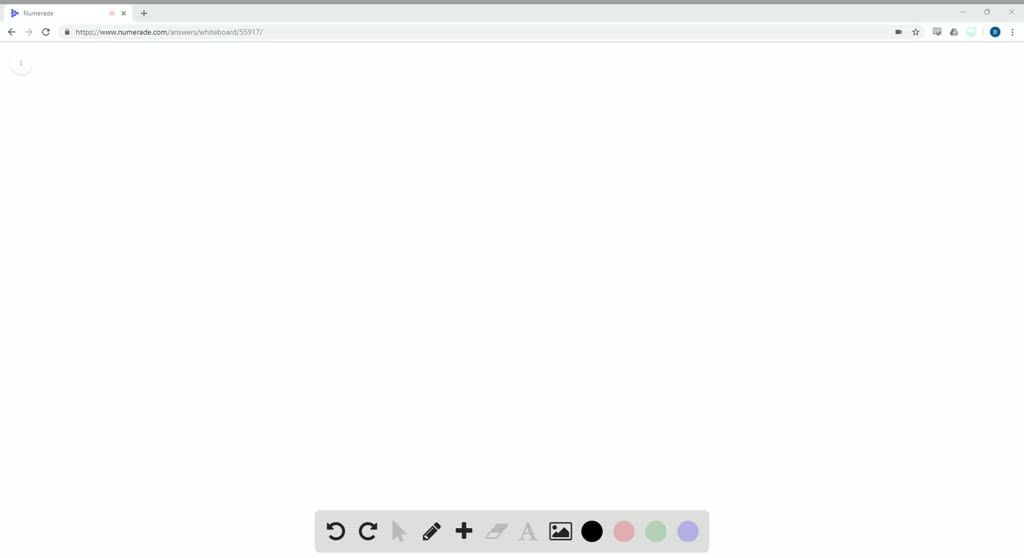A web browser window is displayed on a computer screen. The current tab shows a blue triangle icon pointing to the right, which appears to correspond to a name or title, although the text is blurry and indistinct, possibly reading "New Made" or "Name Made." The browser's address bar is visible, accompanied by standard navigation controls including the back and refresh buttons. On the right side of the address bar, a blue circular icon represents the user profile picture. The main content area is largely empty, featuring a white background with a couple of faint, curvy gray lines at the top left corner just below the back button. At the very bottom of this page, there is a gray rectangular toolbar housing multiple icons: a back button, a forward button, a refresh button, an arrow, a pencil, a plus sign, a portrait, a black circle, a pink circle, a green circle, and a light purple circle on the far-right. Additional obscured icons are also present but not clearly identifiable.